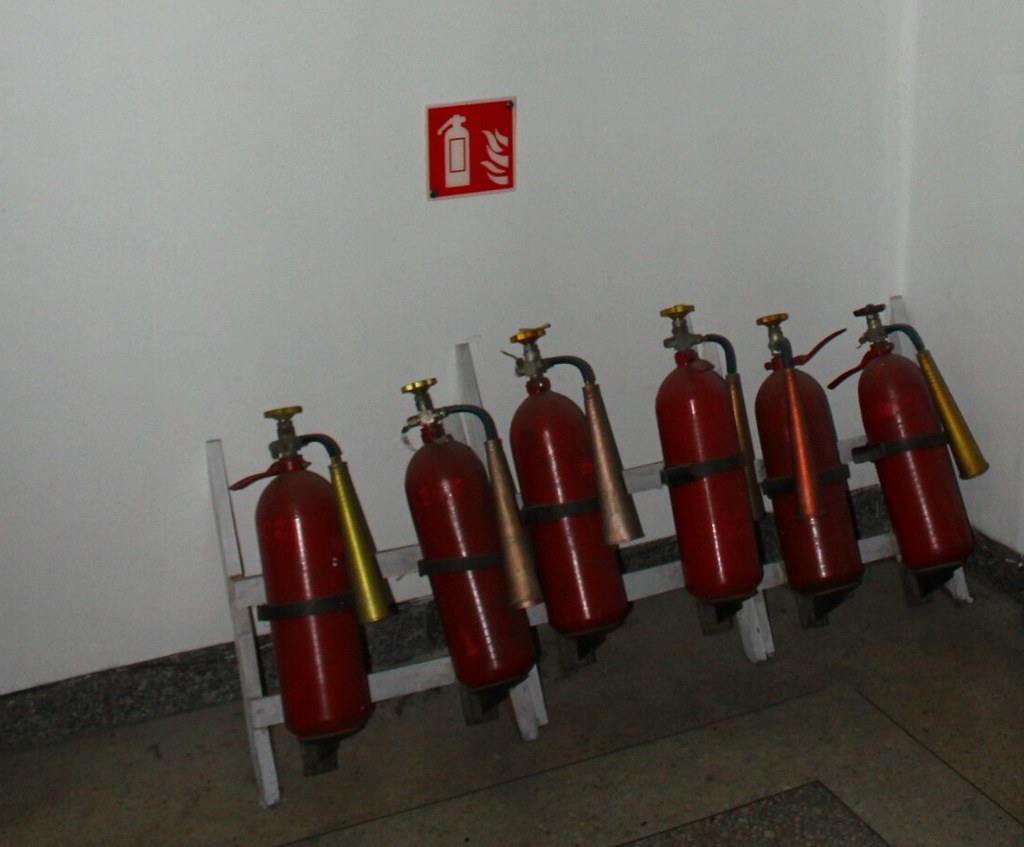The photograph captures a dimly lit corner of a room with polished concrete flooring that continues up slightly as a skirting. The white walls form a neat backdrop, converging in the corner where the focal point lies—a row of six red fire extinguishers neatly mounted on a bracketing system resembling the rungs of a ladder. Each extinguisher features a nozzle and dark red canisters with yellow handles. Above the extinguishers, a prominent square sign with a white border features fire extinguisher and flame symbols in white against a red background, indicating the safety equipment's purpose. The extinguishers are aligned against the rear white wall, slightly varying in height due to their propped arrangement on the rail.